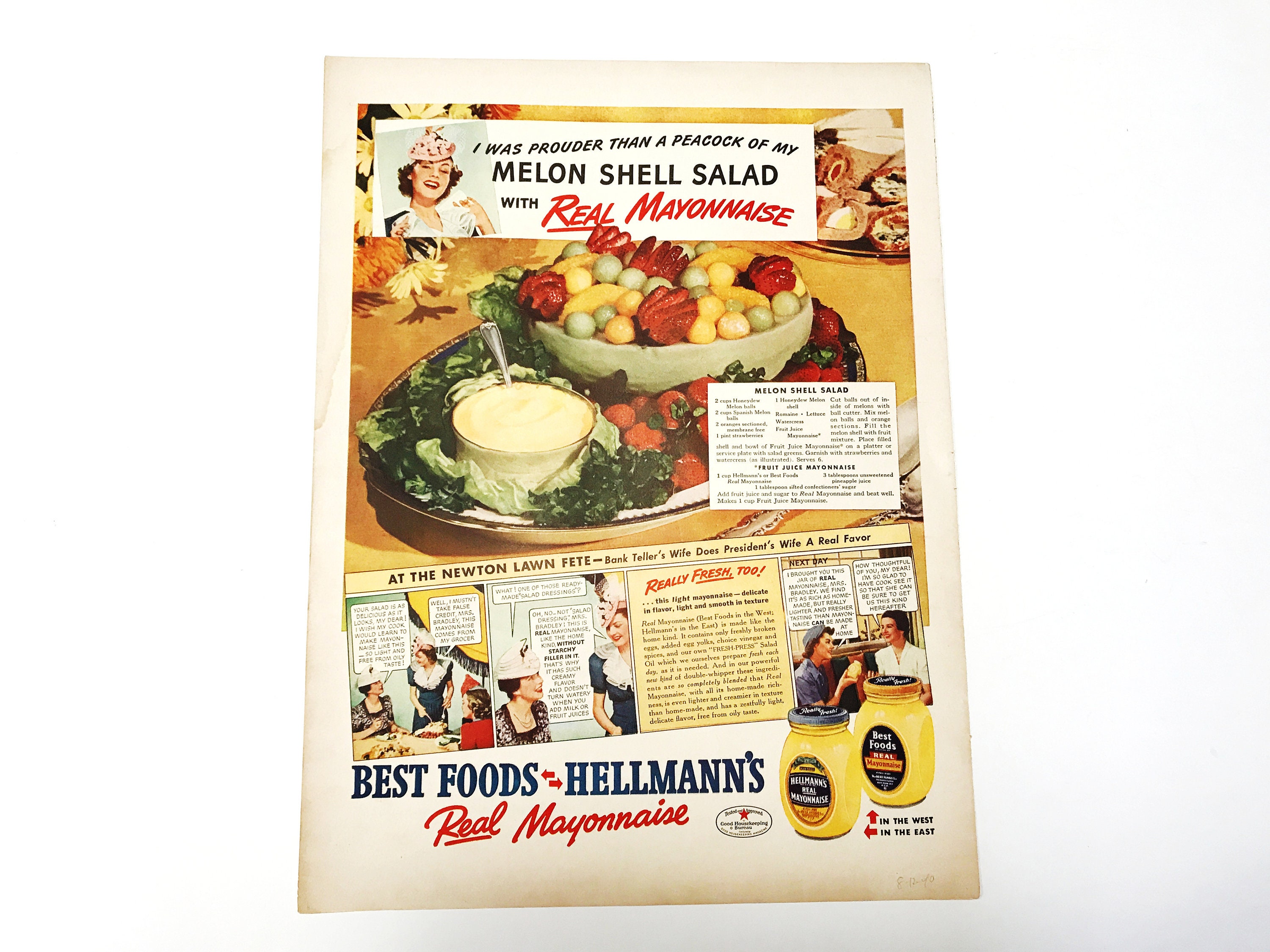This vintage full-page magazine advertisement for Hellman's Mayonnaise, reminiscent of the 1950s, is brimming with retro charm. At the top, a colorful and realistic drawing of a lady boasts, "I was prouder than a peacock of my melon shell salad with real mayonnaise." Below this, there's a vibrant photograph featuring a honeydew melon bowl filled with melon balls, artfully presented on a bed of greens. Accompanying this is a small bowl of mayonnaise-based sauce with a silver spoon. To the side, there’s a square inset displaying the melon shell salad recipe. Further down, the ad includes a comic strip featuring housewives discussing mayonnaise, though the detailed dialogue is not legible. At the very bottom, beside the Good Housekeeping Seal of Approval, appear the words, "Best Foods Hellman's Real Mayonnaise," along with images of vintage Hellman's mayonnaise jars in the bottom right corner. The entire scene is set against a bright yellow background.